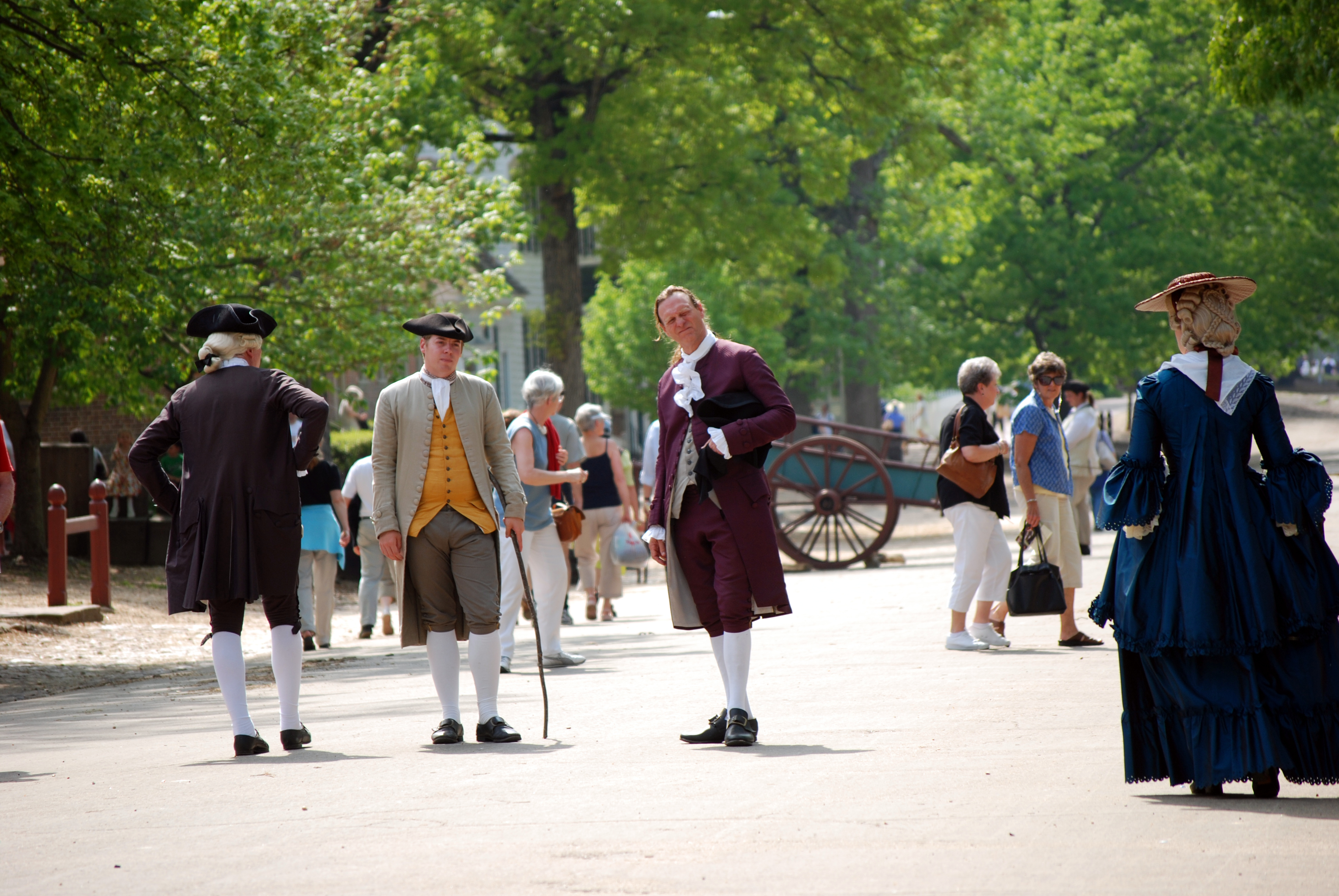In this modern-day photograph taken outdoors in a spacious area, a fascinating blend of the past and present unfolds. The scene features a grove of green trees and a white building in the background, highlighting the bright, sunny day. Scattered throughout, primarily elderly women clad in capri pants and blouses, with purses slung over their shoulders, wander around enjoying the day. However, what makes this image truly unique is the presence of individuals dressed in colonial-era attire, participating in what appears to be a reenactment.

To the right of the picture, a woman stands with her back to the camera, showcasing a long royal blue dress with puffy sleeves and a white scarf draped over her shoulders. Her hair is pinned up in intricate layers beneath a flat tan hat, secured with a maroon ribbon. Near her, facing the viewer, are two men in elaborate period clothing. The gentleman on the right wears a maroon outfit, complete with knee-length pants, white stockings, black buckled shoes, a tailcoat, and a vest. His companion on the left is similarly dressed in a taupe-colored jacket, yellow vest, gray pants, and a black tri-corner hat with a white ruffled shirt underneath.

Further to the left, another man—dressed in darker, black colonial attire with a tri-corner hat, powdered wig, and an elegant black coat—faces away from the camera, adding to the historical ambiance. A wooden wagon, painted teal with brown wheels and rails, rests at the edge of the scene, while wood fence posts frame the composition.

This vivid contrast between the modern tourists and the historical reenactors provides a captivating glimpse into how the past and present can coexist in a single frame.